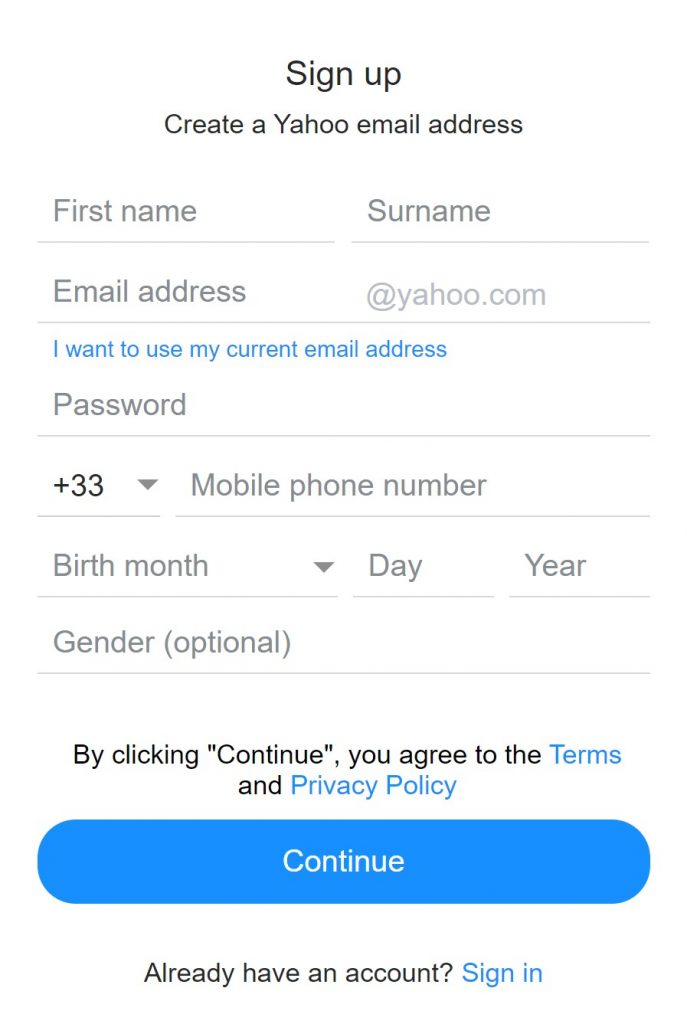The image is a screenshot of a Yahoo registration form in portrait orientation, set against a completely white background. At the upper center, the heading "Sign up" is displayed prominently. The subsequent row prompts users to "Create a Yahoo email address." 

The form begins on the next row with fields to enter a "First name" and "Surname" beside each other. Following this is a row where users input their "Email address." To the right of this field, in very light gray text that blends into the white background, is the domain "yahoo.com." Beneath this, there is an option in blue text, "I want to use my current email address," which redirects users to an alternate form.

The form continues with a field for a "Password." Below this, there's a section for entering a mobile phone number prefixed with the international dialing code "+33" and a drop-down menu to select the country code. For users in America, this would default to "+1."

Further down, there are fields for "Birth month" (with a drop-down menu), "Day," and "Year." There is also an optional field where users can enter their gender. 

At the bottom, there is a disclaimer in black text: "By clicking continue you agree to the Terms and privacy policy," with "Terms" and "Privacy policy" links highlighted in blue. A large "Continue" button follows, which appears disproportionately large relative to the small font size, creating a sense of wasted space.

Finally, at the very bottom, a prompt for existing users reads "Already have an account?" with a blue "Sign in" link to the right. This form is comprehensive, requiring users to enter various details to create a Yahoo email address, with an option for existing account holders to sign in.